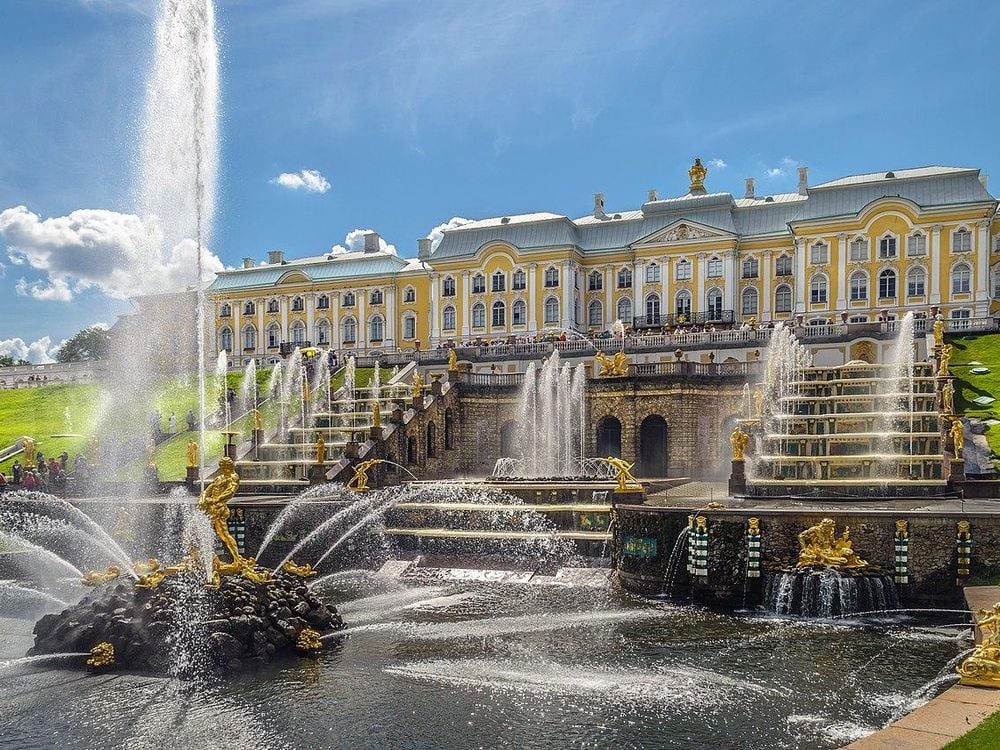This sketch depicts a stunning, grand hotel, likely located in France, with an unmistakably ornate and elegant design bathed in golden and white hues. The massive structure, easily resembling a mansion with potentially over 40 rooms, stands majestically against a background of sunny yet slightly cloudy skies. The hotel's front area bursts with activity, showcasing numerous tourists as tiny specks scattered around the impressive scene.

Descending from the hotel are symmetrical staircases adorned with cascading water fountains, starting from the top and intricately flowing down step by step. The water artistically rises and sprays at each level, ultimately converging into a grand landing that gives way to a vast lake. Within the lake, viewers are treated to a spectacle as water gushes from a golden statue of a man standing on an island in the lake, with six streams arching into the air, creating an enchanting display. Observers are seen marveling at the waterfall both close to the hotel and at various vantage points by the lake, adding to the lively ambiance of the scene.